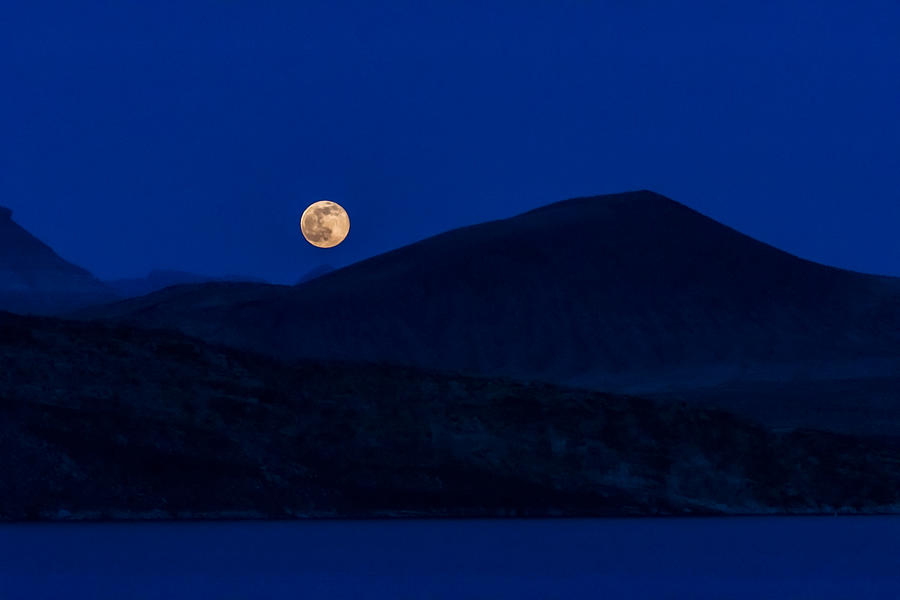This is an artistic night photograph capturing a serene, hilly mountain scene illuminated by a bright, detailed full moon. The entire image is dominated by deep, dark blue hues, with the sky and the landscape seamlessly blending into varying shades of this color. The clear sky takes up most of the upper half of the image, showcasing a prominent moon that stands out in sepia-yellow and gray. The moon rises majestically just above and slightly to the left of the central mountain range, which darkens to a blackish tone and slopes down gently into a flat area at the bottom of the picture.

The foreground features what appears to be a flat, expansive body of water or a snow field, mirroring the blues of the sky. To the right, there is a valley and a lower hill, while the left side of the image is defined by a taller mountain range, adding depth and perspective. The landscape appears to transition into a cliffy area leading down to a potential river or lake. The image, possibly enhanced by a high-quality camera, captures the intricate craters and divots of the moon, making it the focal point against the tranquil, monochromatic backdrop.